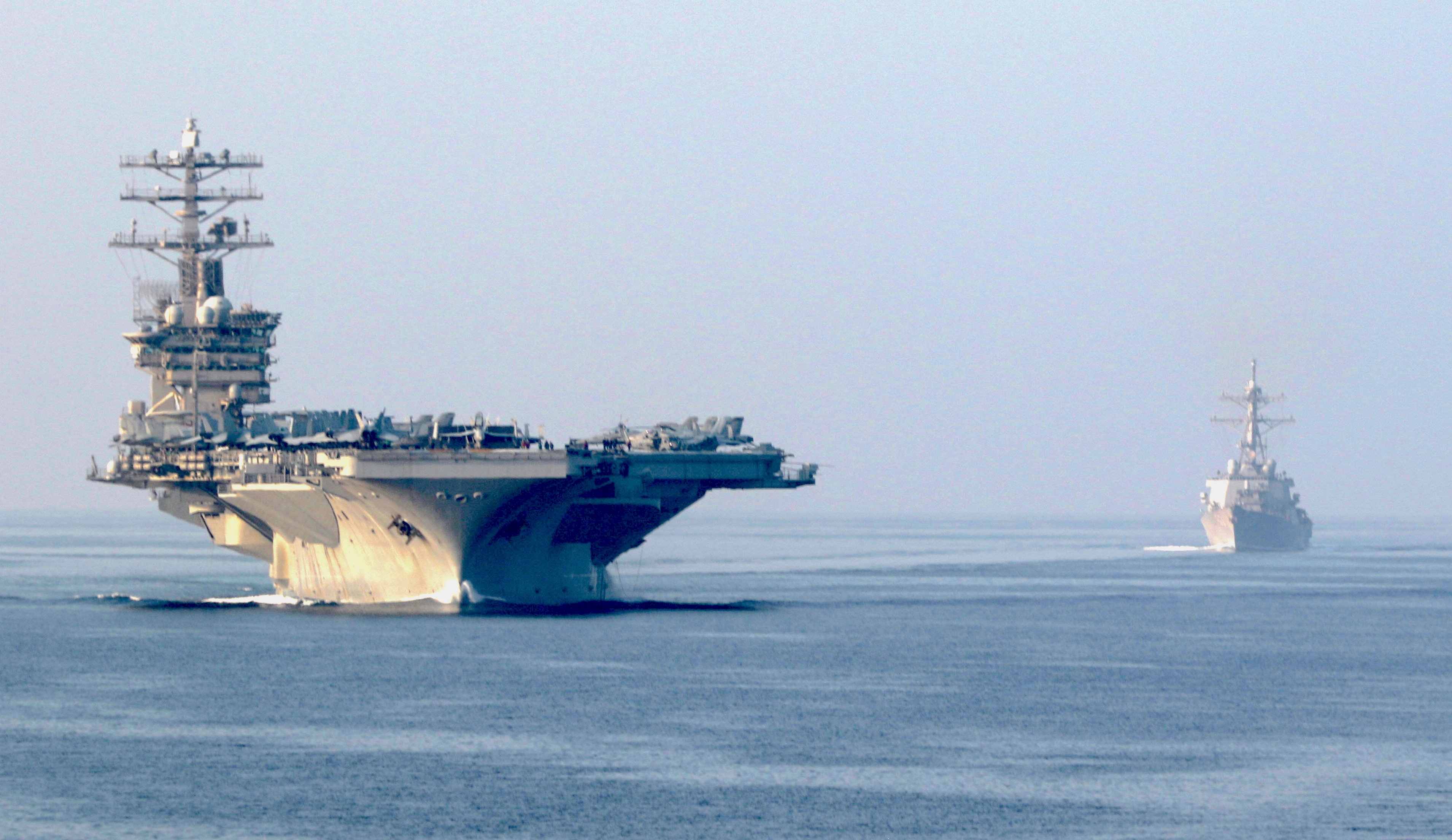The image captures a serene maritime scene dominated by two large naval ships navigating calm, blue waters under a bluish-gray sky. On the left, prominently featured in the foreground, is a colossal aircraft carrier, identifiable by its expansive flat deck, possibly laden with various aircraft and military equipment. The sturdy, T-shaped superstructure rises at the rear of the carrier. To the right and farther in the distance, another smaller vessel can be observed, distinguished by its less flat, more conventional ship-like design indicative of a working or living naval vessel. Both ships are equipped with towering masts and military-grade structures, yet the absence of visible crew adds a sense of stillness to the overall scene. The water surrounding the ships is notably calm, adding to the tranquil aesthetic of the image.